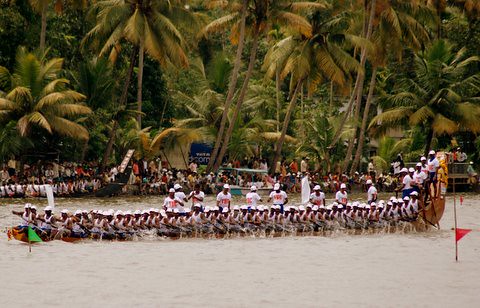The photograph captures a dynamic scene on a tropical body of water, possibly a lake or river, featuring a notably long paddle boat or canoe, measuring around 30 to 50 feet. The boat is filled with numerous rowers, all dressed in white shirts with red trim and white hats, rowing in perfect unison with their paddles perfectly synchronized. The boat features a mid-front section that is low in the water, contrasting with an elevated rear section where some rowers are positioned higher than those at the front. On the boat's right side is a pole bearing a red flag, mirrored by a similar pole with a green flag on the left side. The background reveals a crowd of spectators observing the event, backed by a lush tropical forest with green and brown hues and various high and low palm trees lining the bank. Among the foliage, at least one blue sign is discernible. This vibrant and detailed scene encapsulates a lively and organized aquatic event set against a picturesque natural backdrop.